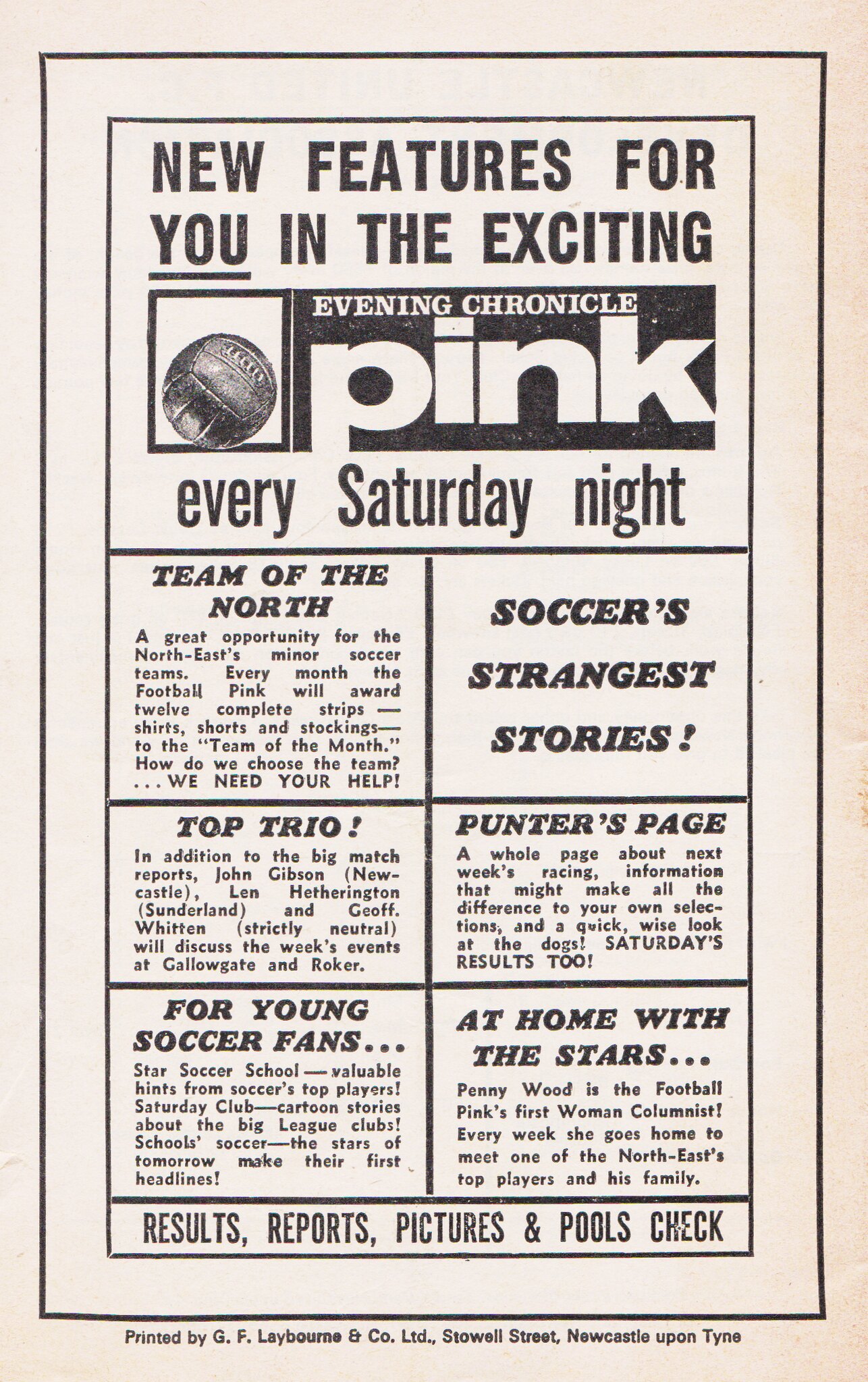The image shows a section of a newspaper, presented in a monochromatic white and black layout, segmented into six small squares with an additional small rectangle above and a larger one below. The upper rectangle displays the bold heading: "New Features For You," with "You" underlined, followed by "In The Exciting" in a lighter font. Below this, in a black box, is the title: "Evening Chronicle Pink," flanked by a symbol resembling a football in a black square to the left. Directly beneath the title, it reads, "Every Saturday Night."

In the six segmented squares below, starting from the top left and moving right, the first reads "Team Of The North" with a short paragraph underneath; the second headline is "Soccer's Strangest Stories!" The second row begins with "Top Trio Title," followed by "Punter's Page," both accompanied by brief paragraphs. The last row features "For Young Soccer Fans..." and "At Home With The Stars...” each with ellipses and a small paragraph. At the bottom of the section, it lists: "Results, Reports, Pictures, and Pools Check."

The entire layout is bordered in black, with black print set against a relatively light pinkish background, emphasizing the soccer-related themes and features within the "Evening Chronicle Pink," published every Saturday night.